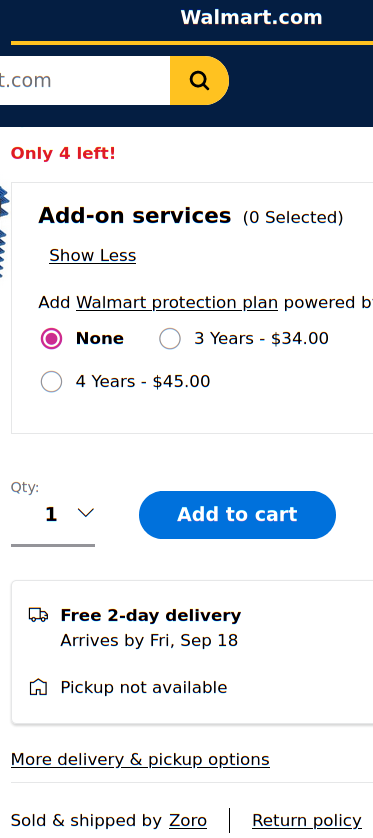The image captures what appears to be a close-up screenshot of a shopping page on Walmart.com. At the top, there is a dark blue section banner with "walmart.com" written in white, located near the top right-hand corner. A yellow line spans horizontally across the banner. On the left side, half of a search bar is visible, ending with a diagonal magnifying glass icon. The search bar's background is also yellow.

Directly beneath this banner, the background transitions to white. In the top left corner, text in red reads "only 4 left!" followed by a larger black font stating "Add-on Services (0 selected)". Below this, the text "Show less" is visible. The next line features a dark blue banner-like font with "one at the top" written on it. Underneath, the text "Add a Walmart Protection Plan powered by [cut off]" is shown.

Continuing down, there are selectable options for protection plans. The word "None" is in bold black, next to a filled pink circle indicating it is selected. Beside it, an unselected white circle with the option "3 Years - $34". Following that is another unselected white circle with "4 Years - $45".

Below these options, "QTY: 1" is displayed with an adjacent drop-down box. To the right is a blue horizontal cylindrical button with "Add to Cart" written in white within it. Beneath this button, a side-view image of a delivery truck is shown with the text "Free 2-Day Delivery, Arrives by Friday, September 18th" in bold black. Below the truck image, a line drawing of a house indicates "Pick up not available". At the bottom of the image, the text "More delivery & pickup options" is underlined.

This detailed view offers a comprehensive look at the shopping options and additional services available for a specific item on Walmart.com.